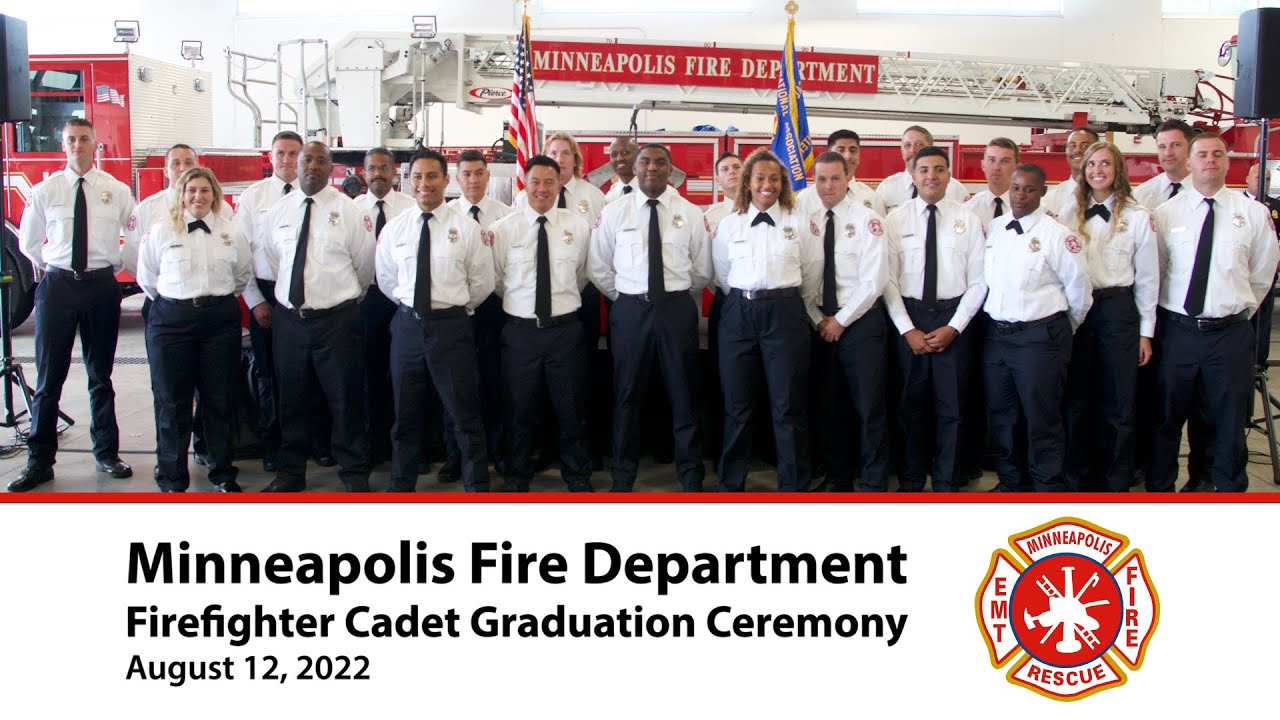The rectangular photograph captures a formal group portrait of multiple graduates from the Minneapolis Fire Department Firefighter Cadet Graduation Ceremony on August 12, 2022. The image is divided into two sections: the top two-thirds dedicated to the photo of the cadets and the bottom one-third featuring a white banner with black text providing details about the ceremony.

In the photograph, the male cadets are dressed in white long-sleeved shirts with black ties, while the female cadets wear similar white shirts but with bow ties at the neckline. All the cadets, both men and women, are also outfitted in navy blue pants. They stand in a line, smiling and looking directly at the camera.

The backdrop features a large firetruck partially visible with a red banner overhead that reads "Minneapolis Fire Department" in a star-style font. There are two flags flanking the group: an American flag on the left and a blue flag with white trim on the right.

Centered within the white banner at the bottom of the image is text detailing the event, "Minneapolis Fire Department Firefighter Cadet Graduation Ceremony, August 12, 2022." To the right of this text is a red circular shield featuring white outlines of a fireman’s hat, ladder, hammer, and pick. Surrounding the circle are four triangular sections with red text stating "Minneapolis" at the top, "Fire" on the right, "Rescue" at the bottom, and "EMT" on the left.